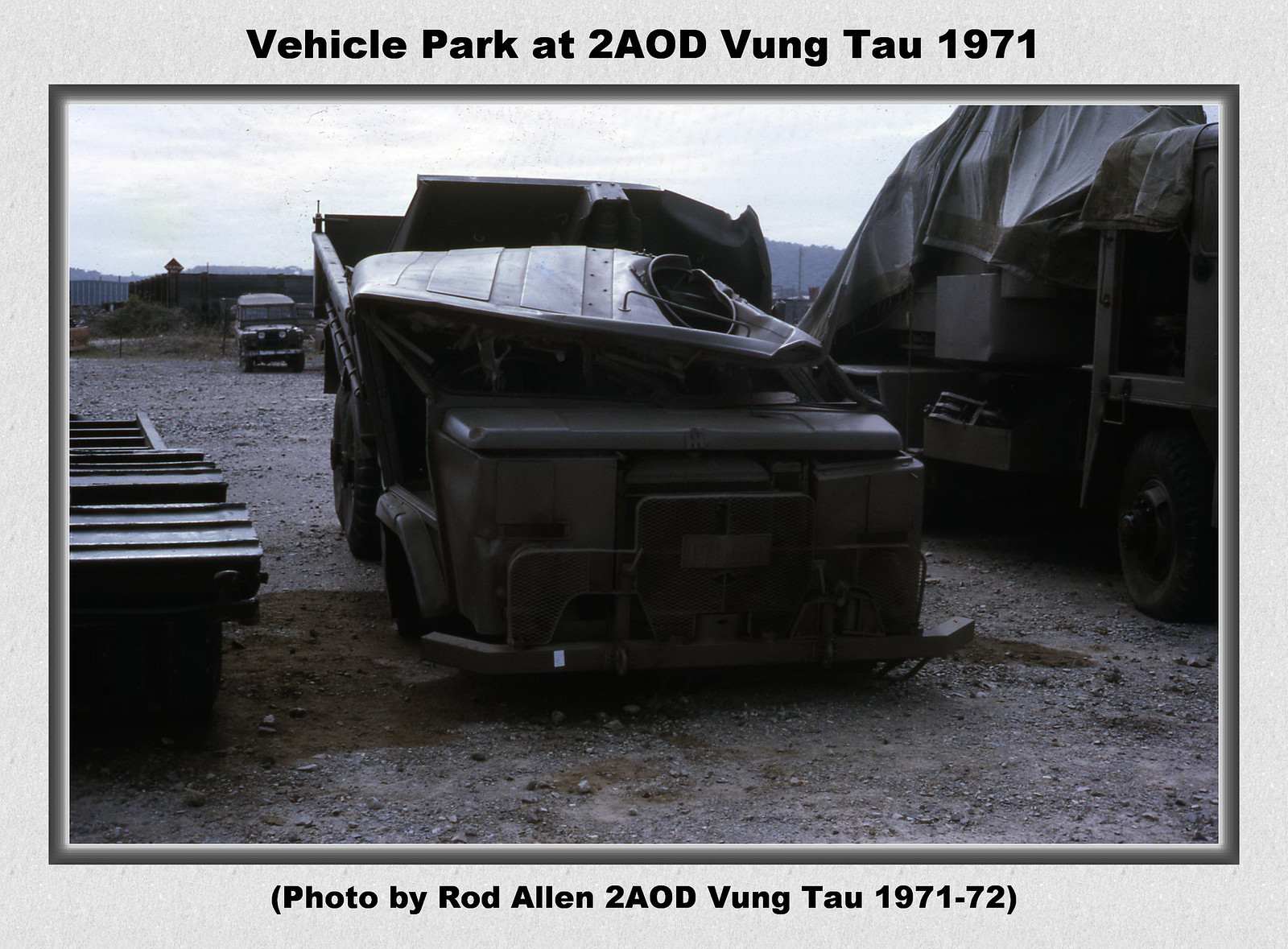The image captures a damaged, grayish, military vehicle with a crumpled top, positioned centrally and extending to the left of the frame. This central vehicle appears square-shaped and has sustained visible damage, indicating it may have been through some kind of incident. The image is titled "Vehicle Park at 2AOD Vung Tau, 1971" at the top and credits "Photo by Rod Allen, 2AOD Vung Tau, 1971-72" at the bottom. 

To the right of the main vehicle is a larger covered truck, likely also military, sheltered under what appears to be a large blanket. On the far left, part of another vehicle is visible, while the bottom section of the image shows some indistinguishable objects that might include a trailer. In the background, there are additional items, including a jeep, and a building standing behind it. The sky is light gray, possibly signaling overcast weather, and there are what look like mountains faintly visible in the distance. The ground is a uniform brown, adding to the overall muted color palette of the old photograph, which emphasizes the dismal and worn look of the military vehicle park at Vung Tau in 1971.